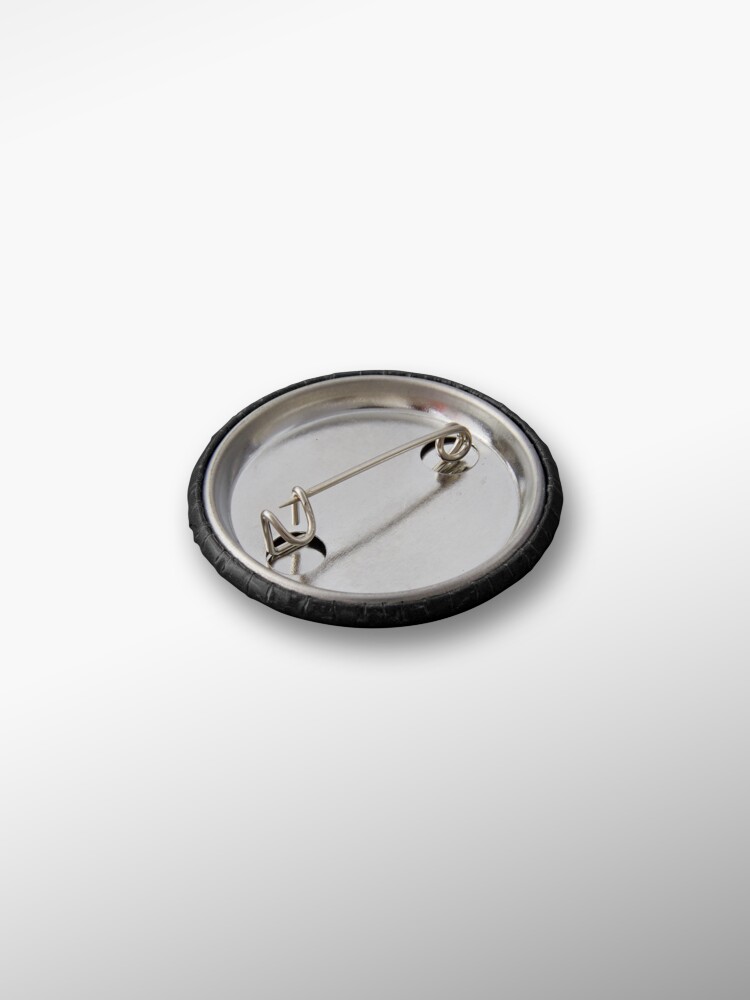The photograph features an upside-down pin badge set against a vertical rectangular background that transitions from a very light gray or white at the top to a slightly darker gray at the bottom. The focal point of the image is the silver, shiny, metallic backside of the pin, which is round and has a black or dark gray outline. The pin is positioned at an angle, with the top right featuring the round base of the pin and the lower left showing the pin clasp in a locked position. The backside of the pin also includes a matte black plastic material beneath the silver cap. The overall background is bright, particularly towards the upper areas, creating a stark contrast with the metallic and dark elements of the pin badge.